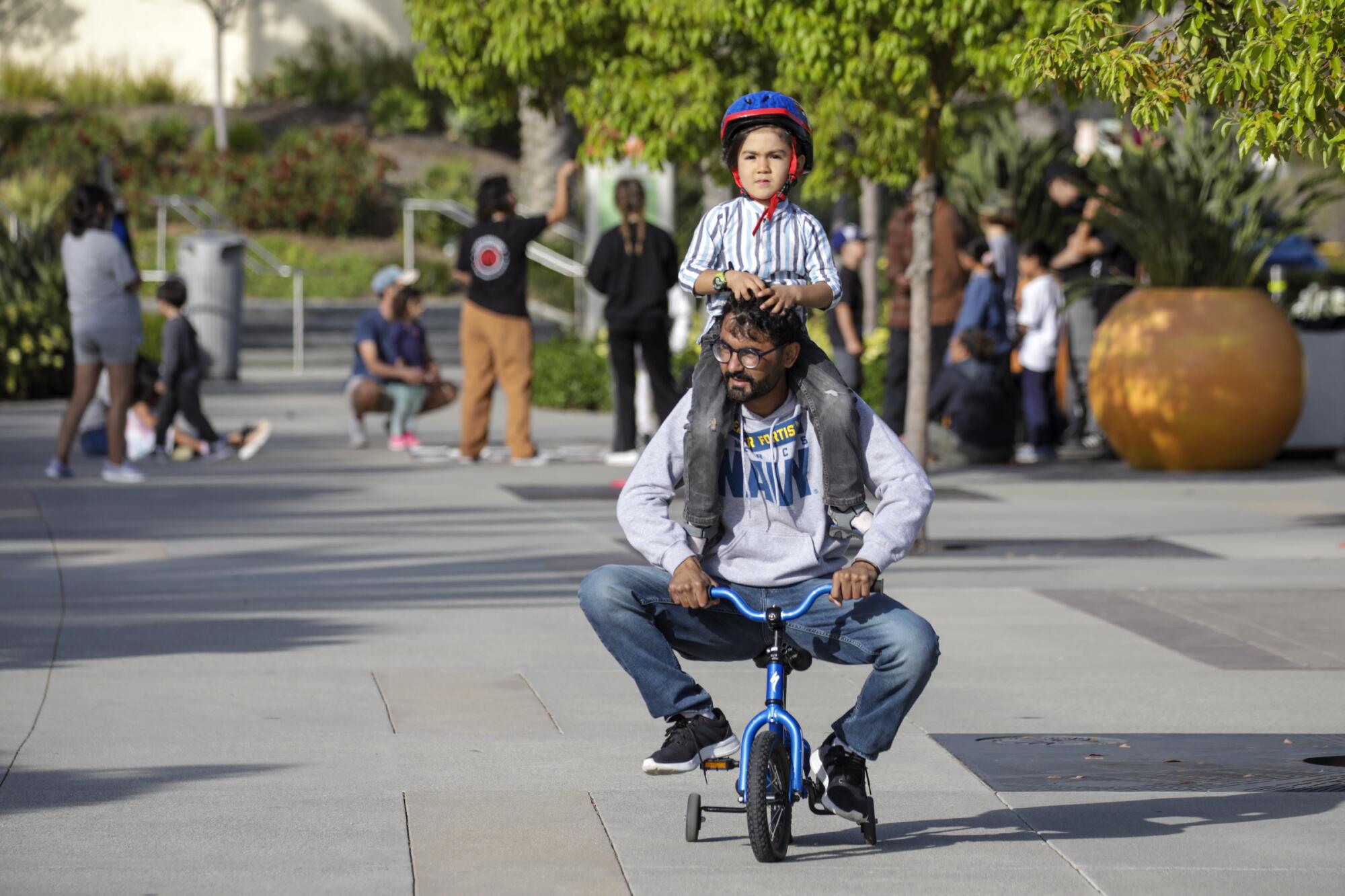In this vibrant and playful outdoor photograph, an African-American man, dressed in a gray sweatshirt with "NAVY" written in blue letters, blue jeans, and black tennis shoes, joyfully rides a small blue tricycle with training wheels on a sunlit concrete path. Perched on his shoulders is a child, who wears a blue helmet with red trim, gray pants, and a striped shirt, their hands playfully resting on the man's head. The scene is set in a park, hinted at by the blurred backdrop of trees and indistinct figures, including other adults and children, enjoying the sunny day. Their positions create charming shadows on the pavement, adding depth to this delightful moment captured in time.